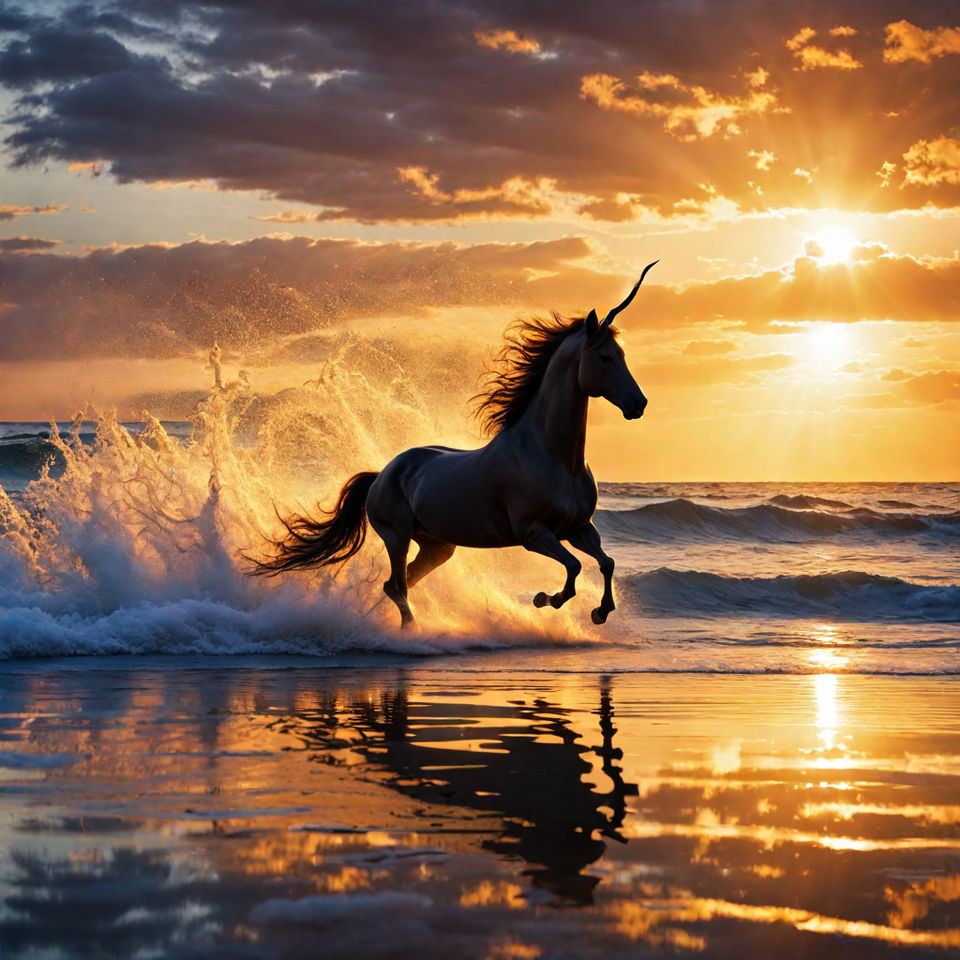This digital painting features a unicorn galloping majestically out of the surf at a wide ocean beach. Centered in the middle of the image, the unicorn, depicted with a slightly crooked horn and light-colored body, dashes toward the right with its mane and brown tail flowing behind it. The water churns and splashes high behind the unicorn, creating frothy white waves. The wet sand at the bottom of the image mirrors the unicorn's dynamic reflection, adding to the sense of motion and depth. A breathtaking sky stretches across the top of the image, bathed in golden sunlight peeking through clouds on the right. This yellowish light blends into shades of pink, blue, and darker gray clouds, creating a dynamic and ethereal atmosphere. The sun, appearing as a round ball with rays streaming outward, casts a luminous glow over the entire right side of the painting, contrasting with the blue ocean waves on the left. This harmonious blend of elements—reflected wet sand, splashing surf, and a radiant sky—creates a mesmerizing and vividly detailed scene.